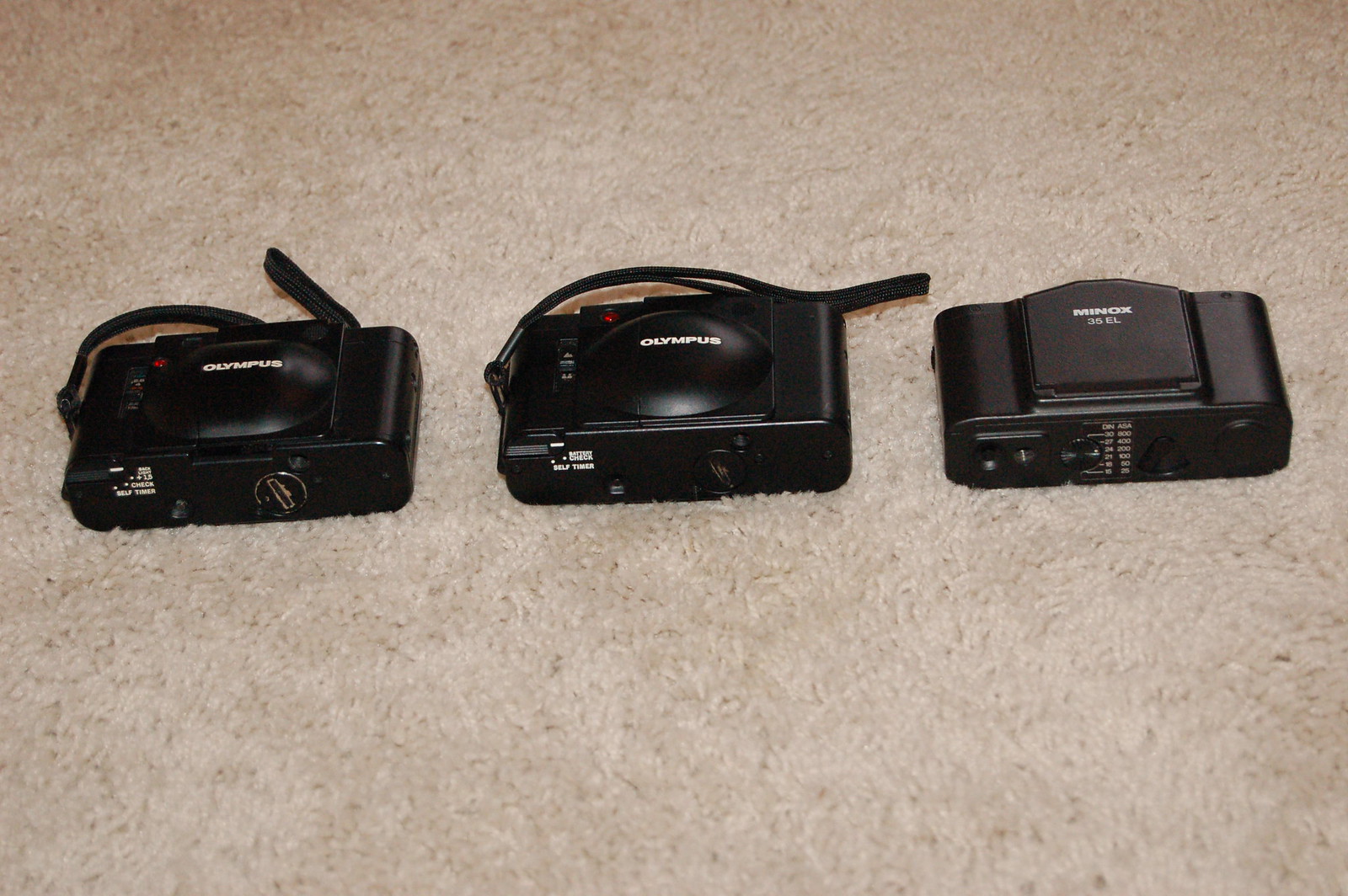The digital photograph captures an indoor scene featuring three vintage film cameras positioned horizontally on a light beige, low-end carpet. The two cameras on the left are identical black Olympus models, featuring a square shape with a raised circular area on top, and 'Olympus' printed in white. These cameras appear without lenses, showing lens caps instead, and have straps extending upward and behind them. The third camera on the right differs slightly in design, being a Minox 35EL, also in black. It has a more rectangular shape with a grip area and lacks the circular bump seen on the Olympus cameras. Despite the subtle differences, all three cameras are displayed prominently in the almost center of the photograph. The image appears to have been taken with a flash, as evidenced by the slight reflections on the camera bodies. Additionally, the bottoms of the cameras reveal markings, including 'self-timer' and various settings like ASA, particularly on the knobs of the Olympus cameras.